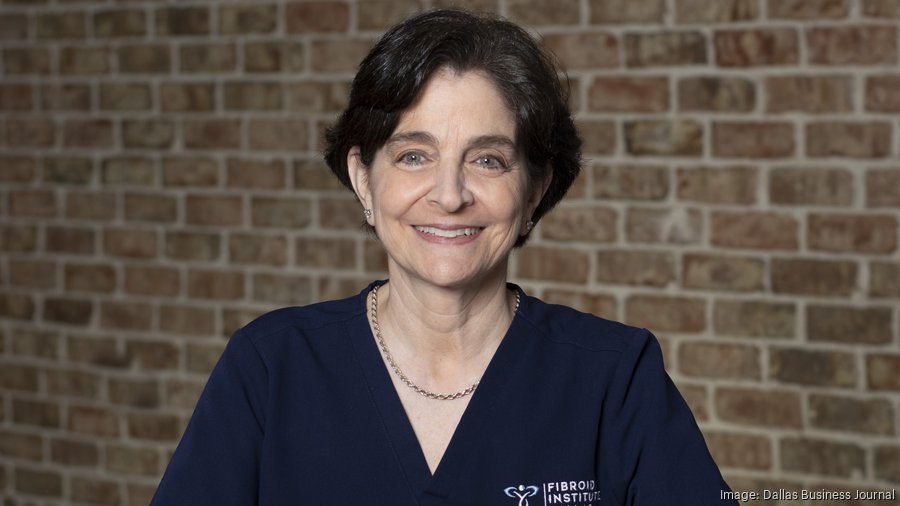In the image from the Dallas Business Journal, a woman stands centrally posed, smiling warmly at the camera, against a backdrop of a red and brown brick wall with white concrete mortar. Her black hair is parted in the middle, tapering off towards her ears, complementing her thick, bushy eyebrows and grayish eyes. She appears to be in her early 60s and accessorizes with a pair of earrings and a gold necklace. She is dressed in a navy blue V-neck uniform, with a white logo on the left side that partially reads "Fibroid Institute." The overall lighting highlights her face while slightly blurring the brick wall behind her, creating a professional yet approachable atmosphere.